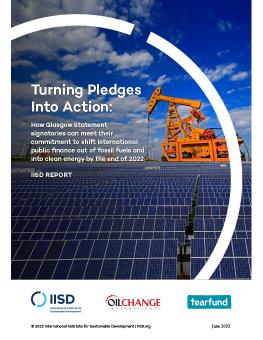The vertically aligned poster, without any border, vividly illustrates the theme "Turning Pledges into Action." Dominating the bottom half are several rows of navy solar panels with crisp, gray lines, neatly arranged in a grid pattern. Stretching from the bottom up to the middle, these panels are set against a backdrop of a partially cloudy blue sky. To the right center of the poster stands a large orange piece of construction equipment, possibly an oil well drill, symbolizing the shift from fossil fuel dependence. Above the solar panels, a semi-circular white design splits at the top, enclosing the bold white text: "Turning Pledges into Action." The text further elaborates, "How Glasgow statement signatures can meet their commitment to shift international public finance out of fossil fuels and into clean energy by the end of 2022," emphasizing this commitment. Below the main image, a circular logo labeled "IISD" sits prominently, accompanied by the slogan "oil change," with "oil" in black and "change" in red. Additionally, in the lower right corner of the poster, a green rectangle with white text reads "Fair Fund."